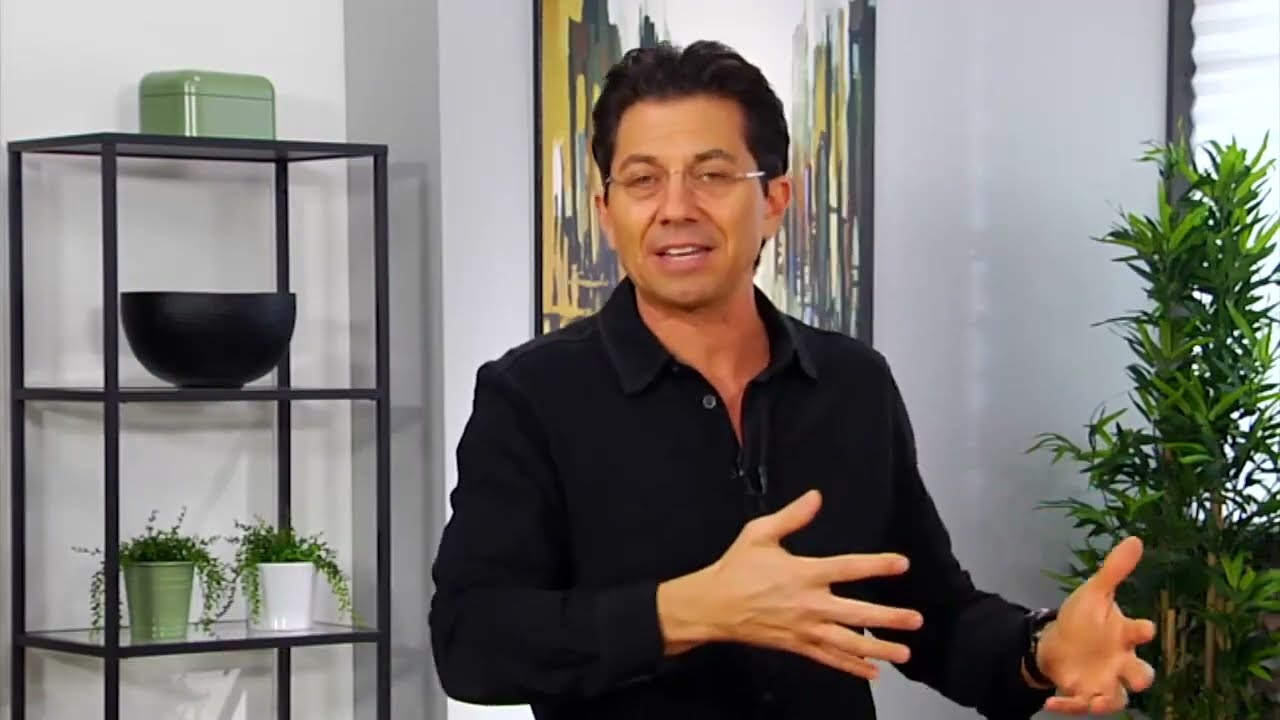The image showcases a man with black hair and glasses, wearing a long sleeve black shirt with slightly short sleeves and a collar, possibly a coat or just a shirt. He stands confidently in the center of the page, his hands extended to his left side, gesturing as if he's presenting or discussing something important. The background appears staged and exceptionally tidy, resembling a set or a perfectly maintained home. To his right is a prominently green plant placed in front of a window with blinds. Behind him, there's a distinctive artwork featuring prominent golden and yellow hues. On the left side of the image, a black-framed shelf with glass levels is visible, housing a variety of items: a light green box on the top shelf, a black bowl on the second level, and two small vine-like plants in white and green planters on the bottom shelf. The whole scene is set against a crisp white wall, further enhancing the orderly and composed atmosphere.